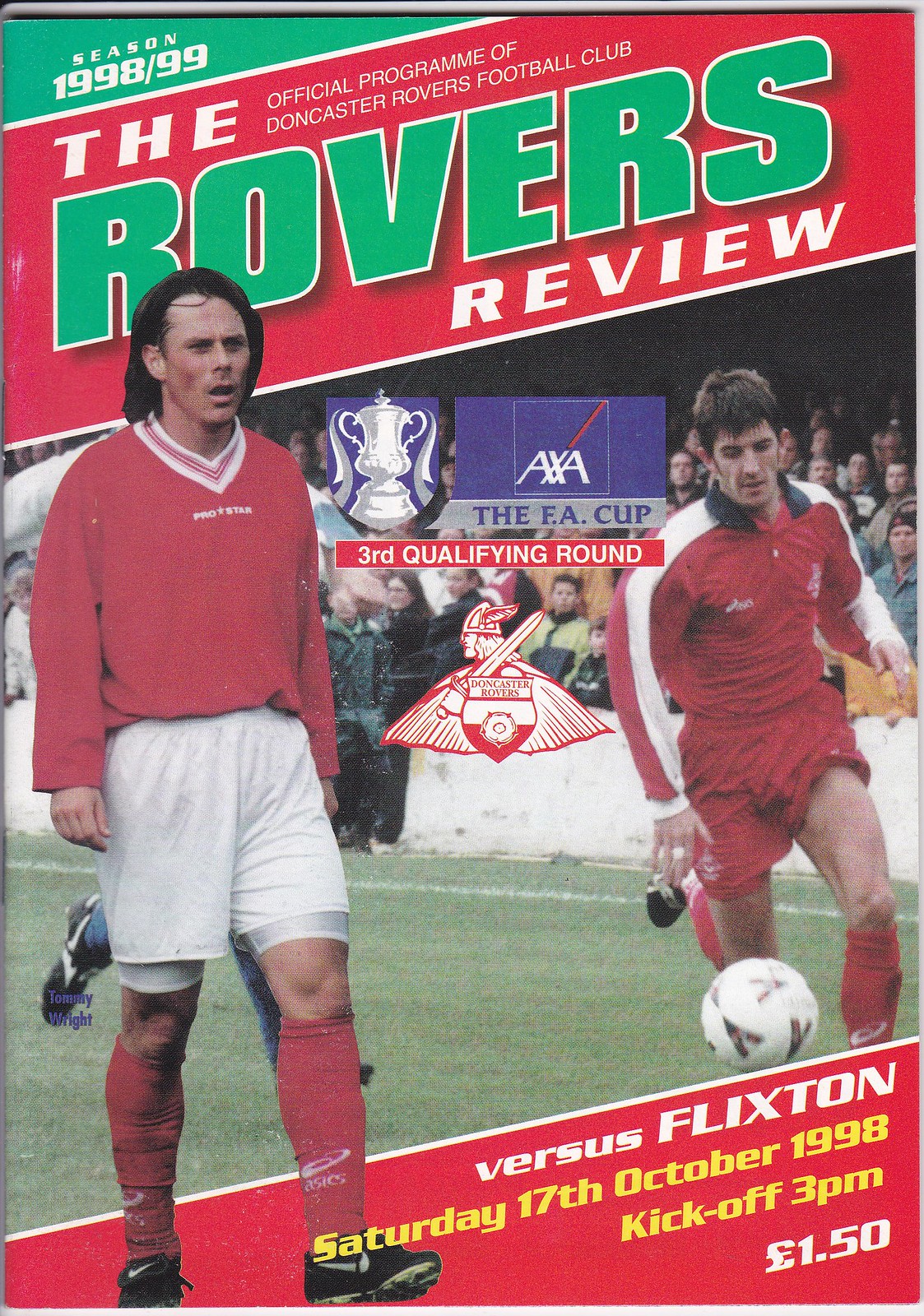This image appears to be the cover of an official matchday program for the Doncaster Rovers Football Club from the 1998-99 season. Dominating the cover is a prominent cutout photograph of a man in the foreground wearing the team's uniform: a long-sleeve red jersey coupled with white shorts, red socks, and black cleats. The title, "The Rovers Review," is displayed in a slightly diagonal orientation across the top with "The" in white letters and "Rovers" in green letters against a red background. Below this, another section reads "Season 1998-99" in white letters against a green background. The lower portion of the cover features a depiction of players actively engaged in a football match with a background crowd, while additional information about the game, including the date ("Saturday, 17th October 1998"), kickoff time ("3pm"), and the price of the program ("euro 1.50"), is neatly positioned in the lower right corner in a slightly diagonal arrangement.